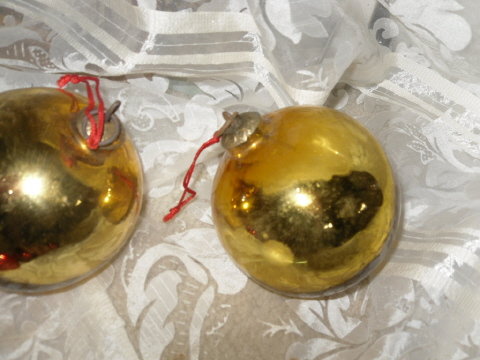The image captures a festive Christmas scene featuring two golden, highly reflective Christmas tree ornaments. These spherical ornaments, capped with gold tops, have red strings attached for hanging, although in this setting they are resting side-by-side on a piece of sheer, shimmery white fabric with satiny designs, possibly stripes or floral motifs. The reflective surface of the ornaments is striking but does not clearly show what they are reflecting. Positioned at 45-degree angles, the ornaments are not suspended but are stationary on the elegant, possibly gauzy white cloth, which adds a delicate and sophisticated background to the festive decorations.